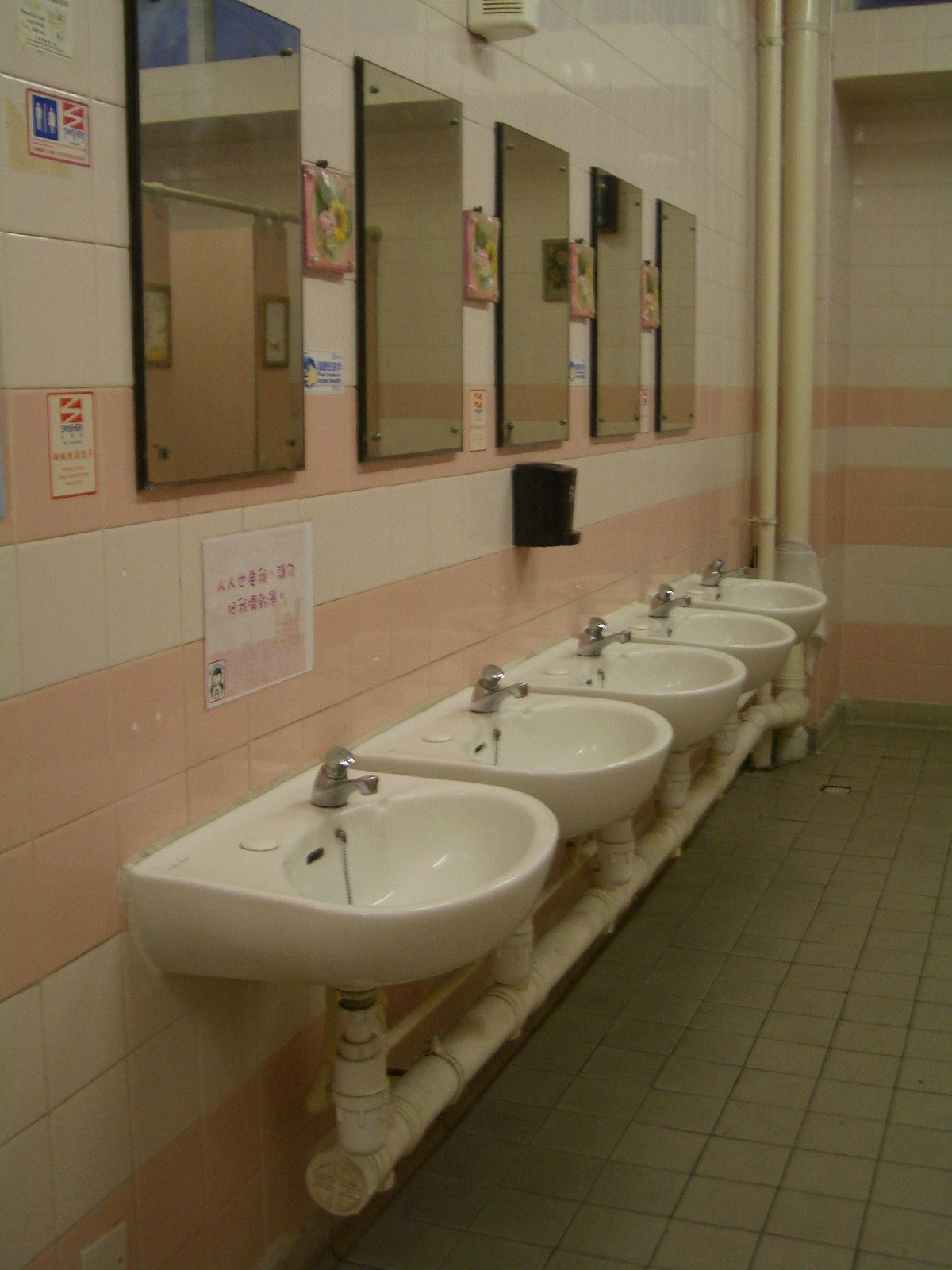This image depicts the inside of a public restroom with a row of five sinks mounted along a tiled wall. The tile design features a series of alternating pink and white lines; halfway up the wall, there's a distinct pink stripe, then a white line, followed by multiple pink and white lines descending towards the floor. Mounted above each sink is an individual mirror, with small pink decorative tiles in between. There's a single black soap dispenser positioned above the middle sink. The sinks are equipped with simple faucets and single levers, and each sink connects to a visible PVC piping system that routes the water into a larger drainage pipe. The floor below consists of smaller, non-glossy grey tiles, resembling cement with etched square patterns. Signs, including one in Japanese, can be seen on the walls.